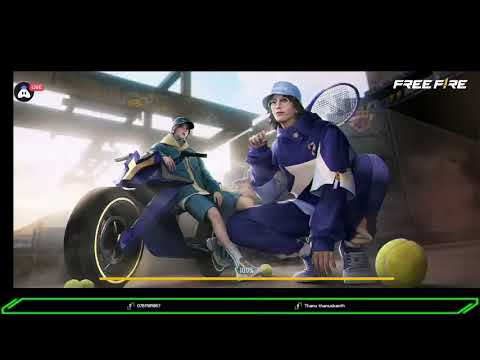The image is a screenshot from the game Free Fire, displayed on a computer with prominent black borders at the top and bottom. The setting resembles a factory with visible big pipes and metal beams traversing the background along with a sky and light source. On the right side, there's a woman squatting with a tennis racket resting on her shoulder. She is dressed in a long-sleeved blue jacket, matching blue exercise pants, and tennis shoes, topped with a blue cap and glasses. A disproportionately large tennis ball is positioned at her feet, appearing prominently in the foreground. To the left, leaning against a purple motorcycle with an extra-large front tire, is another character. This character is dressed in a blue jacket, blue shorts, white tennis shoes, and a blue cap. The bottom of the screen features a green banner with two unreadable names. Additionally, a small "Live" icon is visible on the left side of the image.